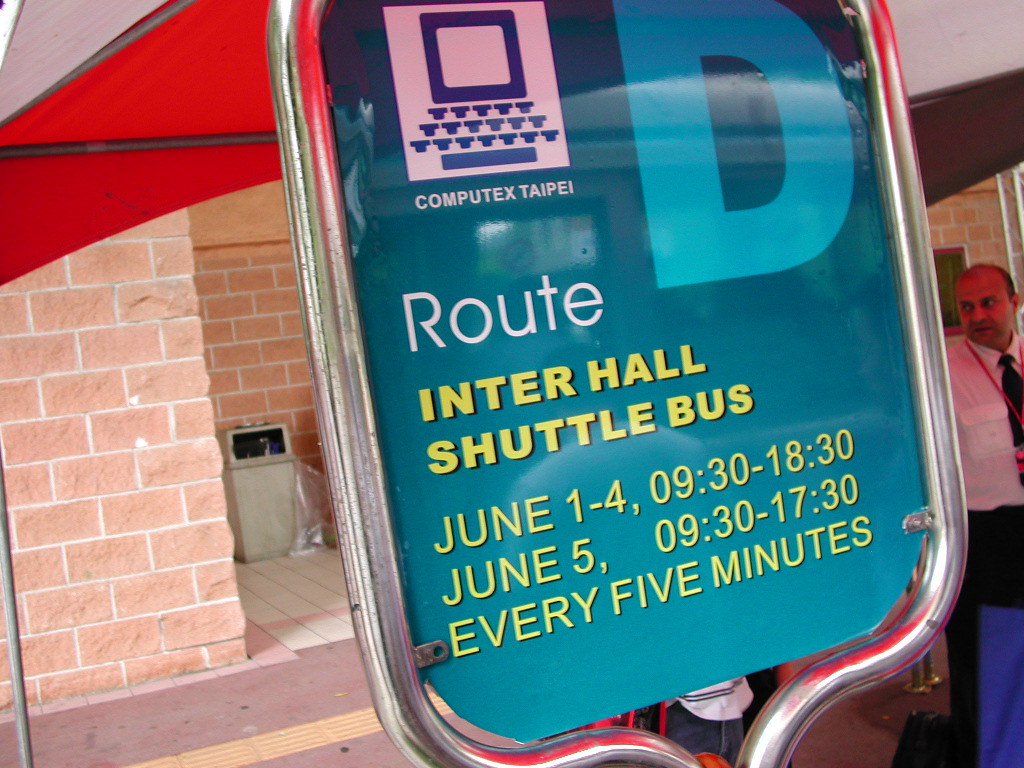The image showcases a detailed scene centered around a sign against the backdrop of a brick building, likely situated at an airport or terminal. Dominating the sign, the large letter "D" is prominently displayed in blue, indicating Route D. Beneath, the text "Inner Hall Shuttle Bus" is highlighted in yellow. It details the shuttle schedule: from June 1 to 4, operating from 9:30 to 18:30, and on June 5, from 9:30 to 17:30, with buses running every five minutes. The top left of the sign prominently reads "Computex Taipei." The sign itself appears to be in dark teal. In the surroundings, a white monitor resembling keyboard keys is visible, alongside a trash can and paved asphalt road. In the distance to the right, a man in a white collared shirt, black tie, and lanyard stands, possibly balding, adding depth to the scene.